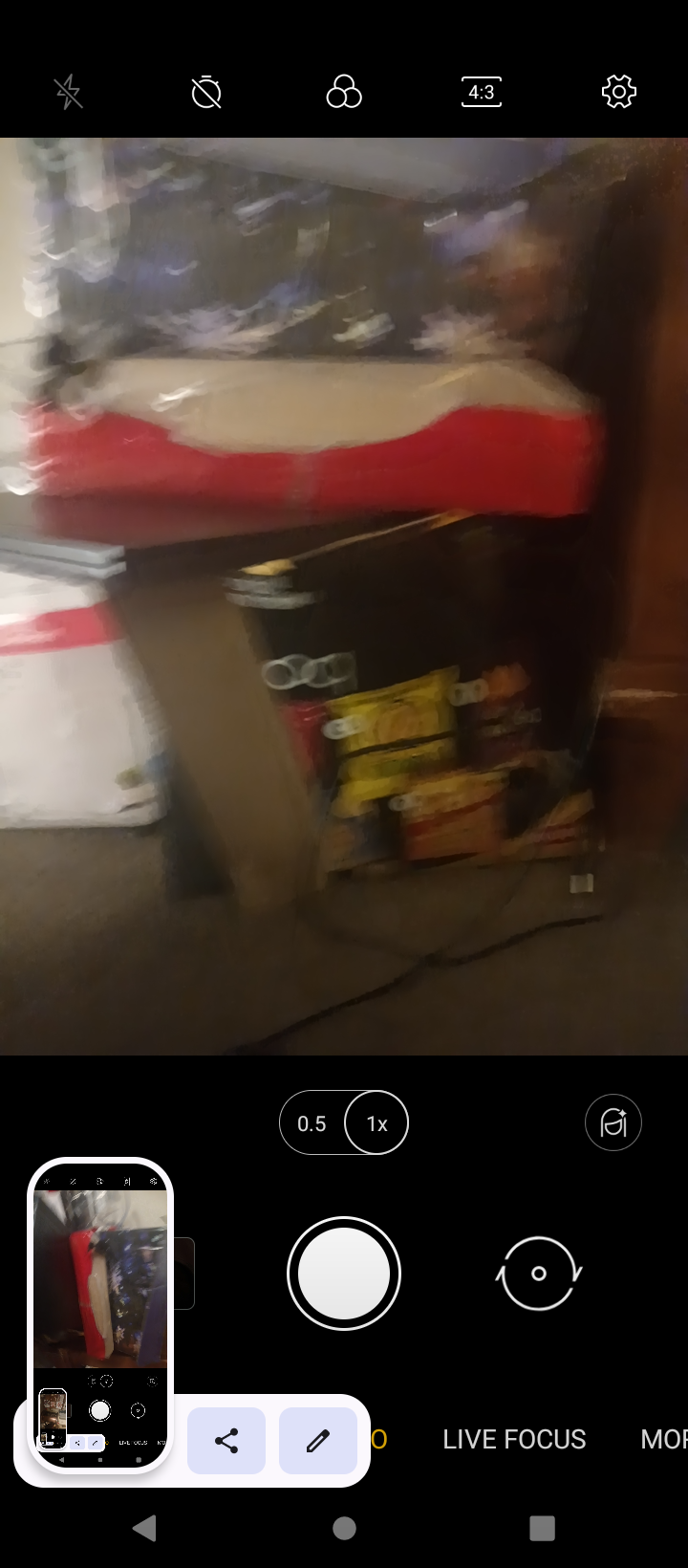This image is a detailed screenshot from a smartphone's camera interface. At the top of the screen, icons representing various camera features are visible within a black rectangular background. These icons include options for adjusting perspective, color settings, general settings, and flash control (indicating whether the flash is on or off).

At the bottom of the screen, various camera controls are displayed. The central white button with a black background is the shutter button used for taking pictures. To its left, there is an icon depicting a circular arrow, signifying the switch between the rear and front cameras of the phone. To the right of the shutter button, a toggle button allows users to switch between 0.5x and 1x zoom levels.

Additionally, within the bottom third of the image, there is a smaller inset image that is a miniature version of the entire screenshot. This "picture within a picture" further emphasizes the camera's interface.

The main section of the screenshot captures what the camera is aimed at—a cluttered and blurred scene of a room. There appears to be a chair, a table with a red box on it, and a bag on the floor. Due to the disheveled nature of the scene and the blurriness, precise details are hard to discern.

Overall, this image is a comprehensive representation of a smartphone camera's interface, concurrently illustrating the scene the camera is capturing at that moment.